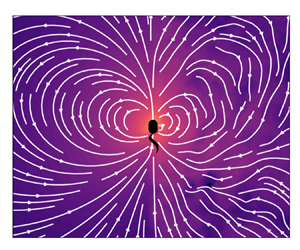This image is an abstract, computer-generated illustration featuring a central black figure resembling a tadpole or sperm. The black silhouette, characterized by an oval body and a squiggly tail, is set against a background that transitions from a glowing orange in the middle to a deep purple around the edges. Surrounding the central figure are irregularly shaped white lines that form spirals and semicircles, emanating outward in a concentric pattern. These lines, varying from squiggly and circular to longer shapes, create a dynamic and intricate design. The white lines wrap around the black figure, giving an impression of wings or an aura, with some converging into the central tadpole-like shape. The overall effect is a vivid, radiating composition with a faint red glow in the center, adding to the visual complexity of the piece.